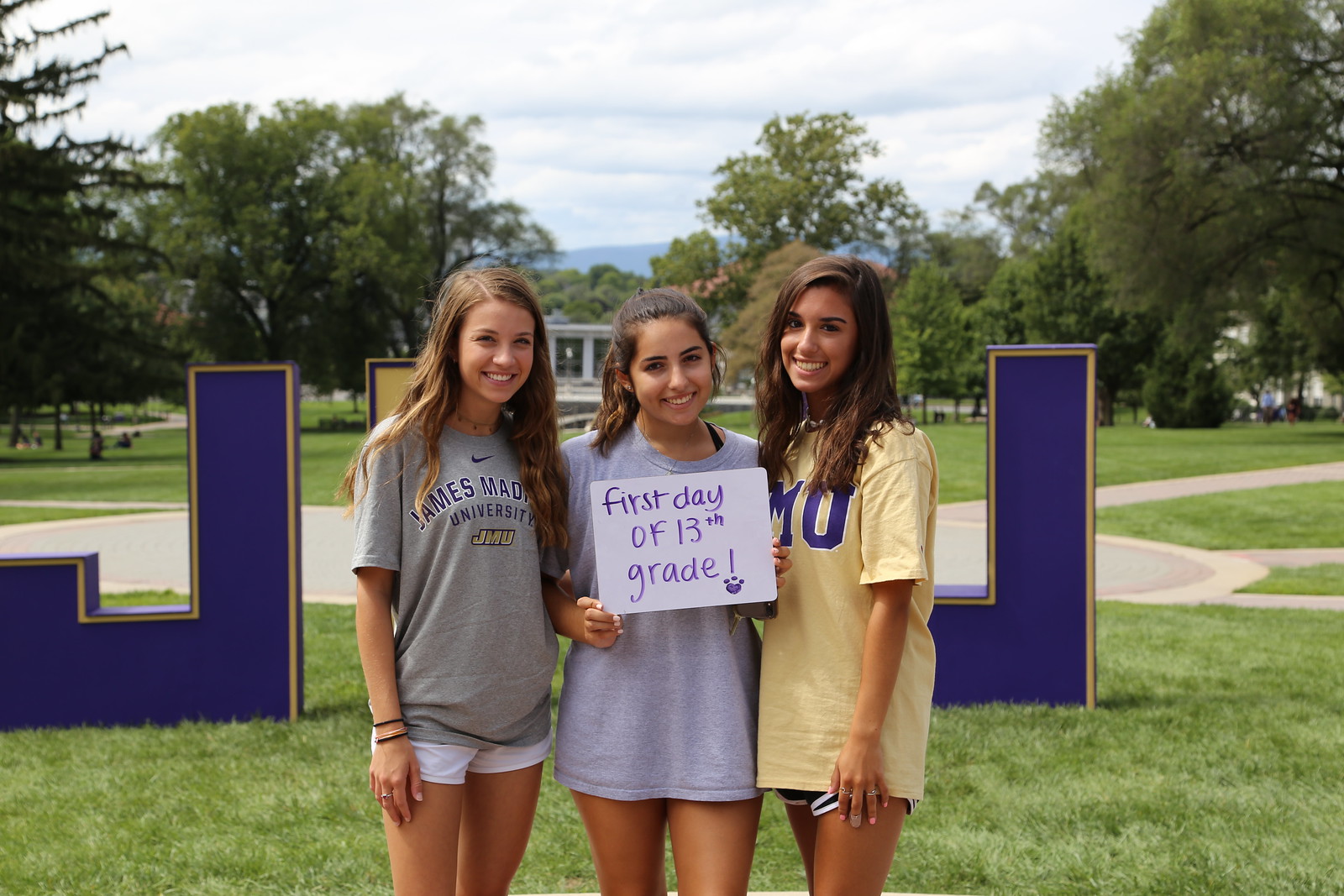In this outdoor, daytime image, three young girls stand side-by-side, all smiling and proudly wearing James Madison University (JMU) shirts, indicating their freshman status. The girl in the middle holds a sign reading "First day of 13th grade," underscoring their humorous take on starting college. The girl on the far right wears a yellow shirt with "JMU" displayed in purple letters, while the other two girls sport gray shirts. The girl on the left is also distinguished by her white shorts. All three have long brown hair. Behind them, a large JMU sign in purple and gold letters stands on a grassy field, with the university campus, numerous trees, and distant mountain ranges visible in the background. The blue sky, mostly adorned with white clouds, contributes to the pleasant and sunny weather. The scene is further complemented by paved sidewalks and a circular pathway, adding to the collegiate atmosphere of the photo.